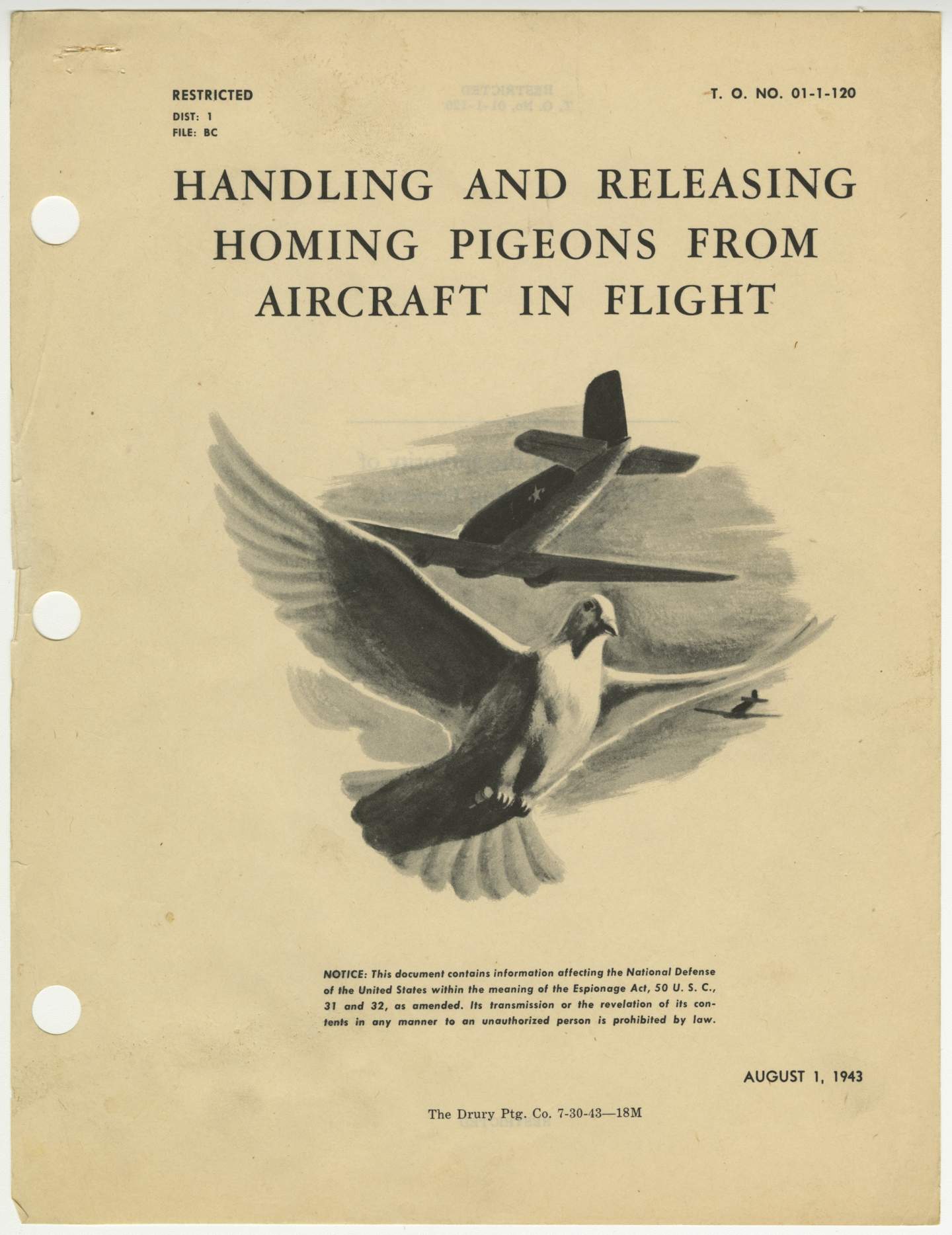The document appears to be a vintage cover page, yellowed with age and showing three hole punches along its left margin, suggesting it was once part of a folder. At the top, in bold black lettering, the word "RESTRICTED" is prominently displayed, indicating its confidential nature. The top left corner also bears the text "DISTRICT ONE FILE BC," while the top right corner is marked with the number "011-120."

Underneath these headings, in large black font, is the title of the document: "Handling and Releasing Homing Pigeons from Aircraft and Flight." Below this title, there is a black and white illustration of an airplane, followed by an image of a pigeon in mid-flight with its wings outstretched and tail feathers spread.

Further down, the notice reads: "This document contains information affecting the national defense of the United States within the meaning of the Espionage Act, 50 USC 31 and 32 as amended. Its transmission or the revelation of its contents in any manner to an unauthorized person is prohibited by law." In the lower left corner, it is dated August 1, 1943, with the additional detail of "The Drury PTG Company 7-30-43-18M" printed below. This document thus pertains to classified information about the use of homing pigeons in aerial operations, crucial for national defense during that era.